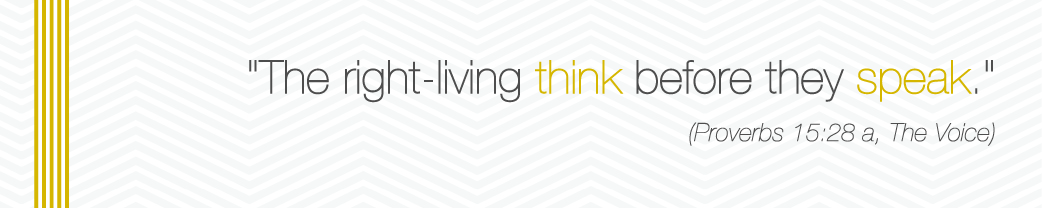This thin rectangular photo poster features a white and blue herringbone background. On the very left, there are approximately five thin vertical gold bars. Centered on the poster, in quotation marks, a Bible verse reads: "The right-living think before they speak." The words "think" and "speak" are highlighted in gold, while the rest of the text appears in light gray lettering. Below the quote, it states in parentheses, "Proverbs 15:28a, The Voice."